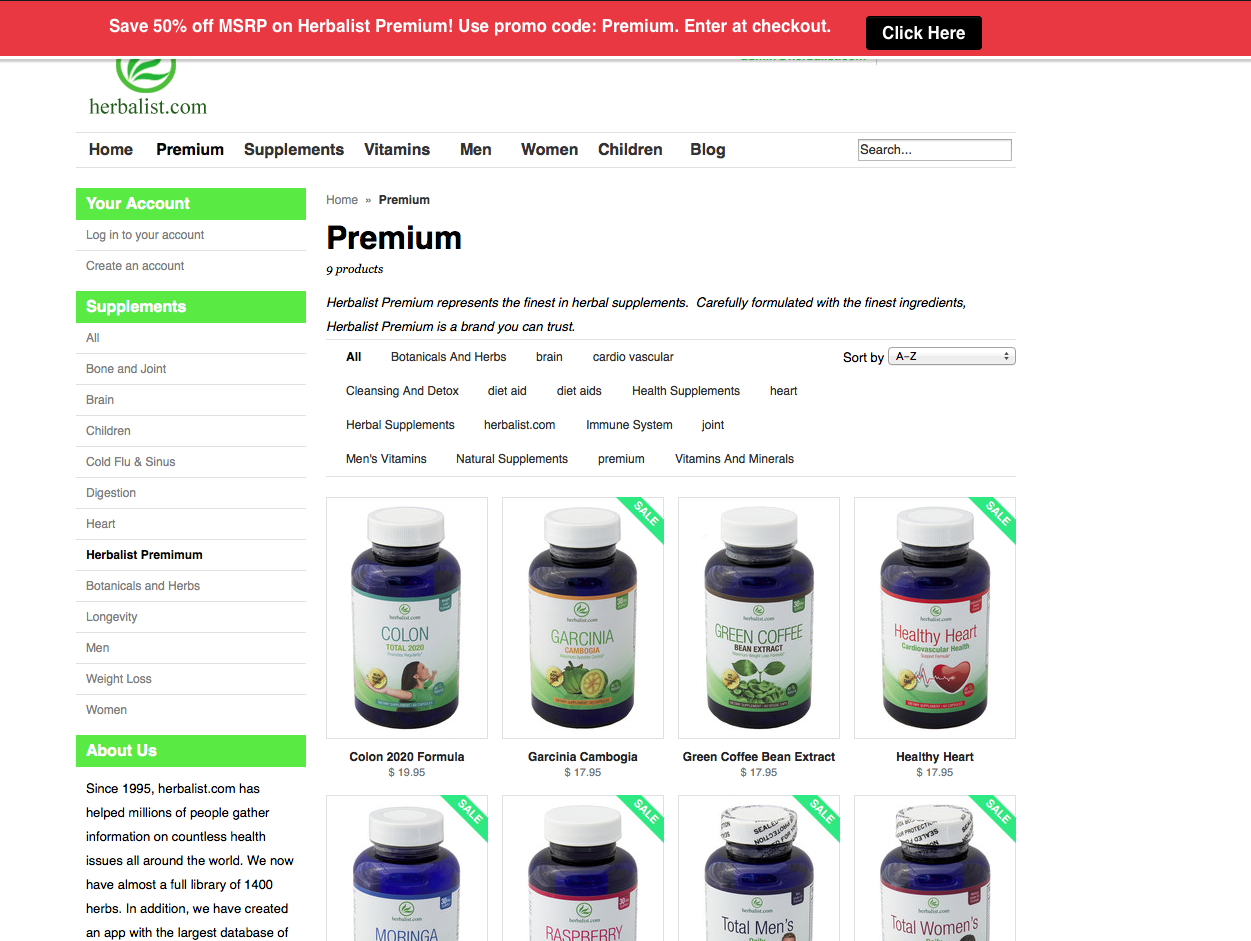This image showcases the homepage of the website "Herbalist.com." At the very top, there is a prominent red banner announcing a promotion: "Save 50% off MSRP on Herbalist Premium. Use promo code 'premium' at checkout." Below this, a black button labeled "Click Here" directs users to take advantage of the offer. The website's name, "Herbalist.com," is displayed next to a green and white logo.

The website's navigation bar offers several sections: Home, Premium, Supplements, Vitamins, Men, Women, Children, and Blog. On the left side of the page, a green sidebar features a section titled "Your Account," with subsections "Log into Your Account" and "Create an Account." Further down, another green bar labeled "Supplements" includes a detailed list of categories: All, Bone and Joint, Brain, Children, Cold and Flu and Sinus, Digestion, Heart, Herbalist Premium, Botanicals and Herbs, Longevity, Men, Weight Loss, and Women.

An "About Us" section highlights the company's history and mission: "Since 1995, Herbalist.com has helped millions of people gather information on countless health issues around the world. We now have a nearly full library of 1400 herbs." It also mentions the creation of an app with the largest database, though the rest of the text is cut off.

In the main content area, there is a section titled "Premium" displaying multiple vitamin and supplement products. Featured items include bottles labeled Colon, 2020 Formula, Garcinia Cambogia, Green Coffee Bean Extract, Healthy Heart, Moringa, and Raspberry. This array showcases the variety of supplements the website currently offers.